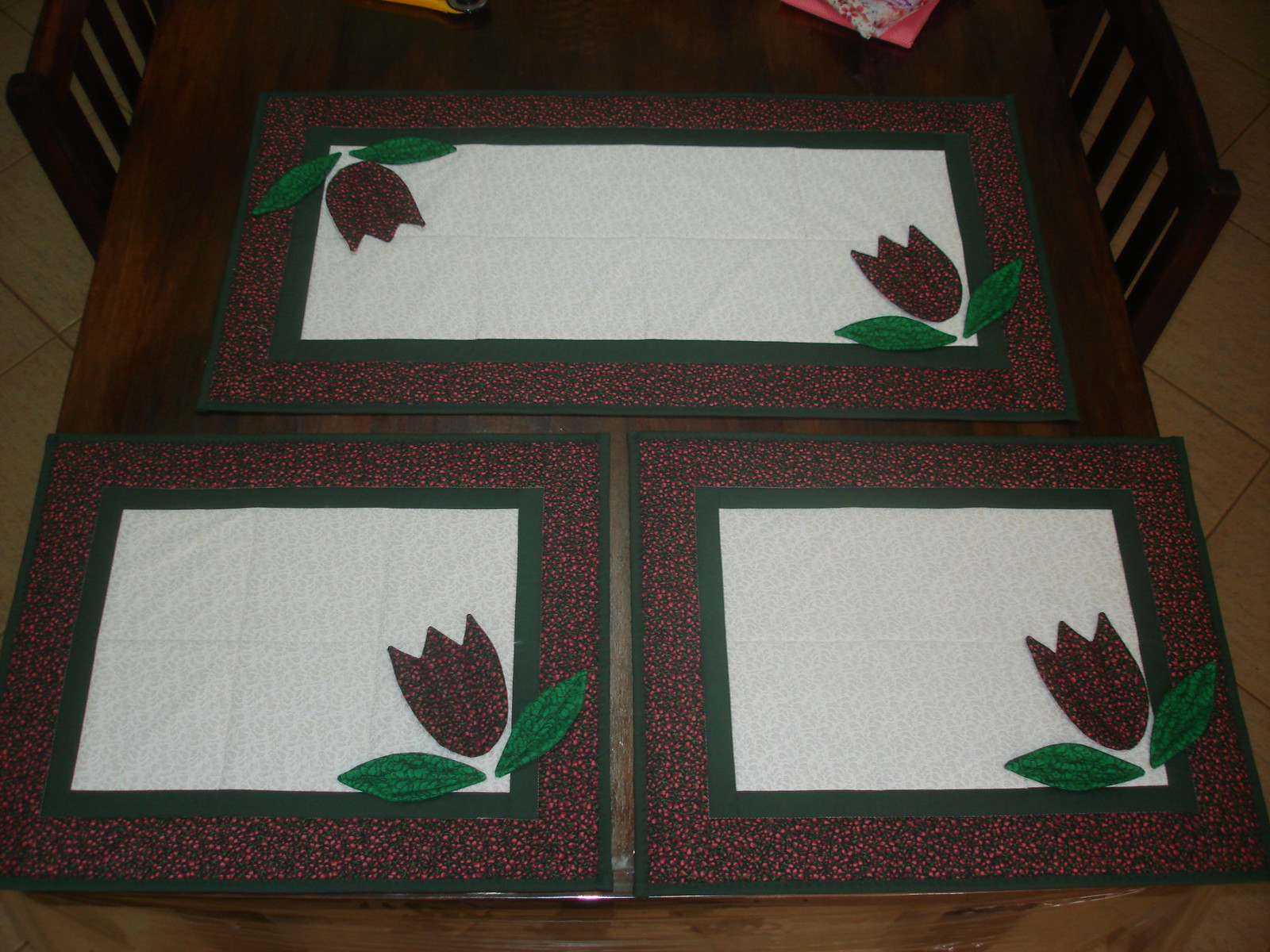The photograph, taken from above in low lighting, captures a dark brown wooden dining table with two matching wooden chairs barely visible at either side. Resting on the table are three embroidered placemats and a longer table runner, each featuring a harmonious floral design. These items are meticulously crafted with a central white square framed by multiple borders: an inner green border, a red and black speckled band, and a final dark green rim. A striking red and black speckled tulip with two green leaves occupies one corner of the square on each placemat, delicately perched against the inner green border. The two square placemats lie side by side at the bottom of the image, while the longer runner, featuring two tulip motifs at diagonally opposite corners, is positioned above them. The wooden texture of the table's surface and the tiled floor visible beneath complete the warm and homely scene.